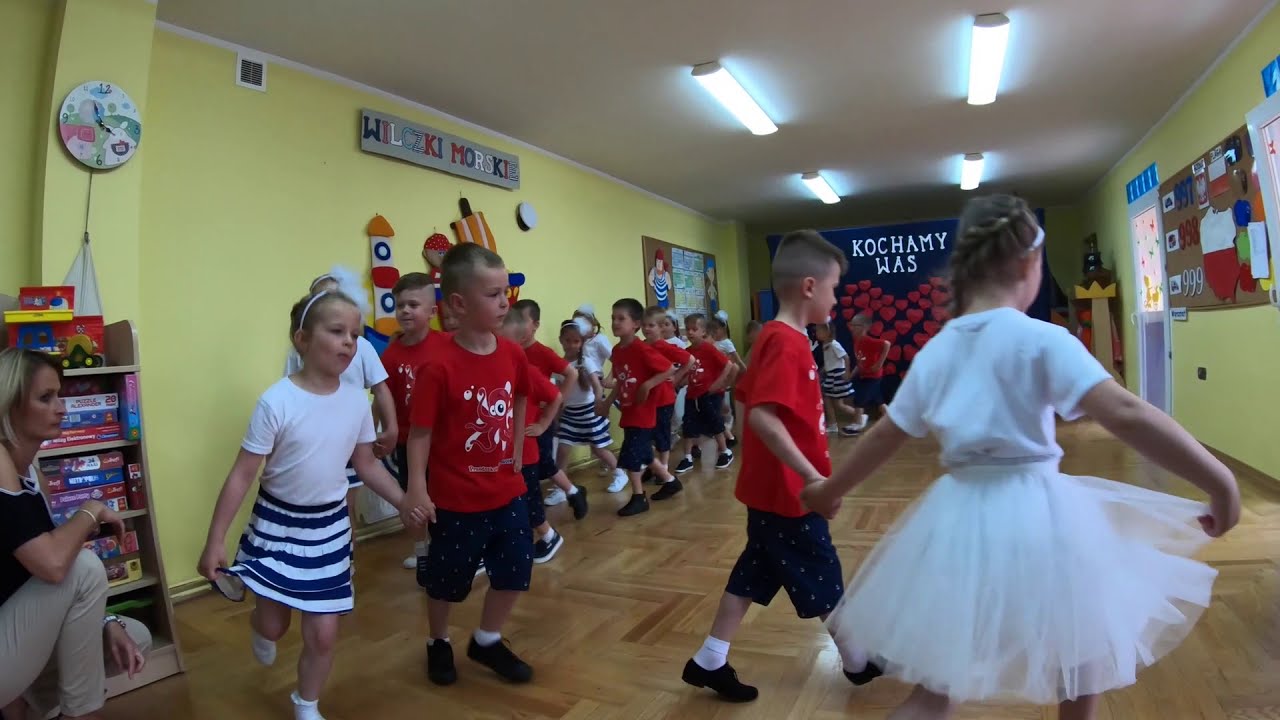This photograph captures a lively classroom scene, likely in a kindergarten or preschool, with walls painted a vibrant yellow adorned with various educational signs written in a foreign language. The ceiling is white, fitted with four tube lights. In the back right corner, a blue screen decorated with heart-shaped balloons stands out prominently, adding a festive touch.

A group of young children is the focal point, engaged in what seems to be a circular dance or a game. The boys, in red T-shirts with cartoon designs and black shorts patterned with white polka dots, hold hands with the girls, who are dressed in white short-sleeve T-shirts and blue and white striped skirts. The leading girl stands out in a white tutu and matching T-shirt, reminiscent of a ballerina. Both boys and girls wear white socks with black shoes for the boys and white shoes for the girls.

The children form a curving line, dancing and moving joyfully. An instructor stands to the left of the room near a book rack, guiding the children through their activity. The scene is vibrant and dynamic, capturing a moment of youthful energy and learning in this brightly decorated classroom.